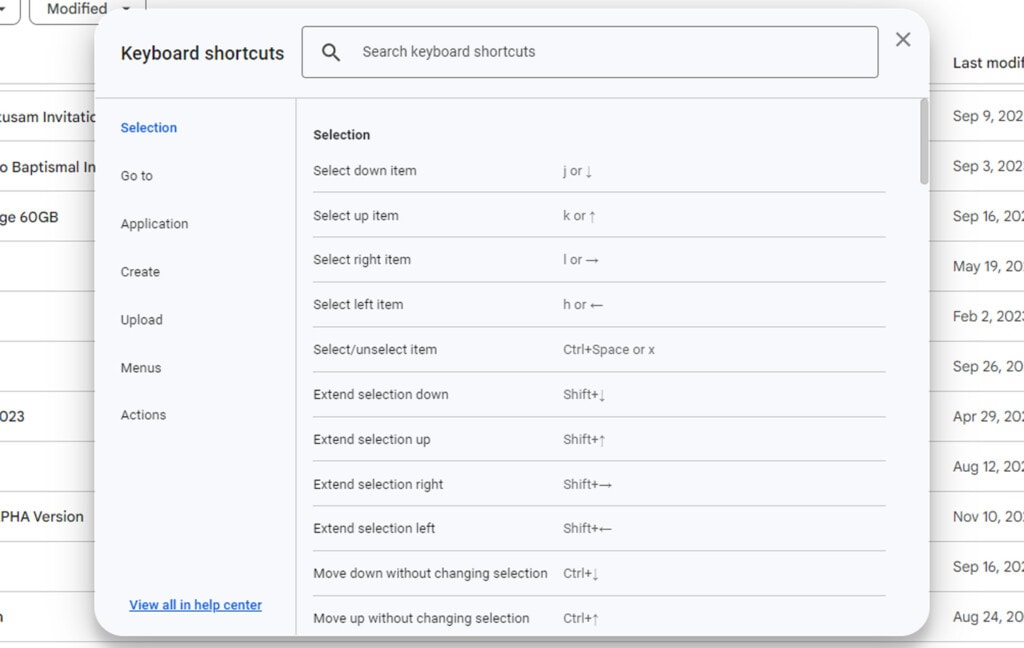The image is a horizontally rectangular screen capture from a computer, displaying a prominent pop-up window in the center. This pop-up window, titled "Keyboard Shortcuts," features a search field at the top left for finding specific shortcuts. An 'X' icon is located in the top right corner, which can be clicked to close the window. 

Beneath the "Keyboard Shortcuts" title, on the left side of the pop-up, there's a vertical list of categories for different types of shortcuts: "Vertical Selection" (highlighted in blue to indicate it is currently selected), "Go To," "Application," "Create," "Upload," "Menus," and "Actions." At the very bottom of this list, a blue link labeled "View All in Help Center" offers additional help resources.

The right side of the pop-up provides detailed information about the "Vertical Selection" category. It lists various keyboard shortcuts for navigating and selecting items: 
- "Select Down Item"
- "Select Up Item"
- "Select Right Item"
- "Select Left Item"
- "Select/Unselect Item"
- "Extend Selection Down"
- "Extend Selection Up"
- "Extend Selection Right"
- "Extend Selection Left"
- "Move Down Without Changing Selection"
- "Move Up Without Changing Selection."

Each function is paired with its corresponding keyboard shortcut key, which is displayed to the right of the description. 

In the background, behind the pop-up window, some additional line item information is partially visible on the left and right sides of the screen.